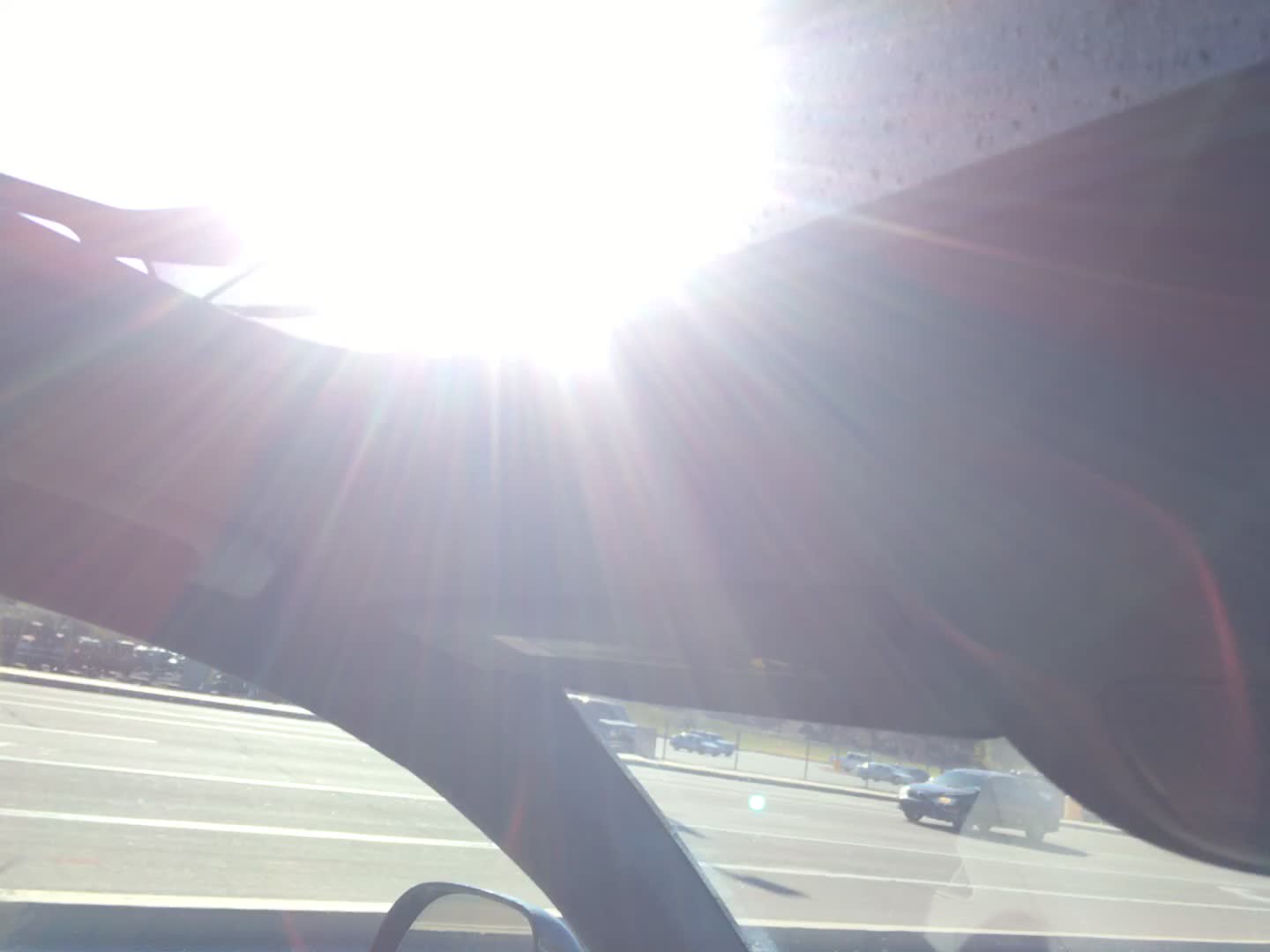This photograph, taken from inside a car through a partially opened sunroof, features the sun as its most prominent element. Positioned in the upper third of the frame, the radiant sun bathes everything in a brilliant, almost overwhelming light, creating distinct rays that enter the car. The intense brightness casts a hazy glow, blurring the details around. Through the sunroof and windshield, a variety of vehicles are visible, including a blue car and several other cars that appear silver. The scene includes a large parking lot, delineated by a metal chain-link fence, with numerous parked cars. Toward the background, there's a building situated past an open grassy area dotted with small trees. The bottom edge of the photo also captures a glimpse of the car's side mirror, indicating the vehicle might be red. The left and front views through the windows show a black asphalt road with white lines, interrupted by the glow of the sun, making some elements hard to discern.